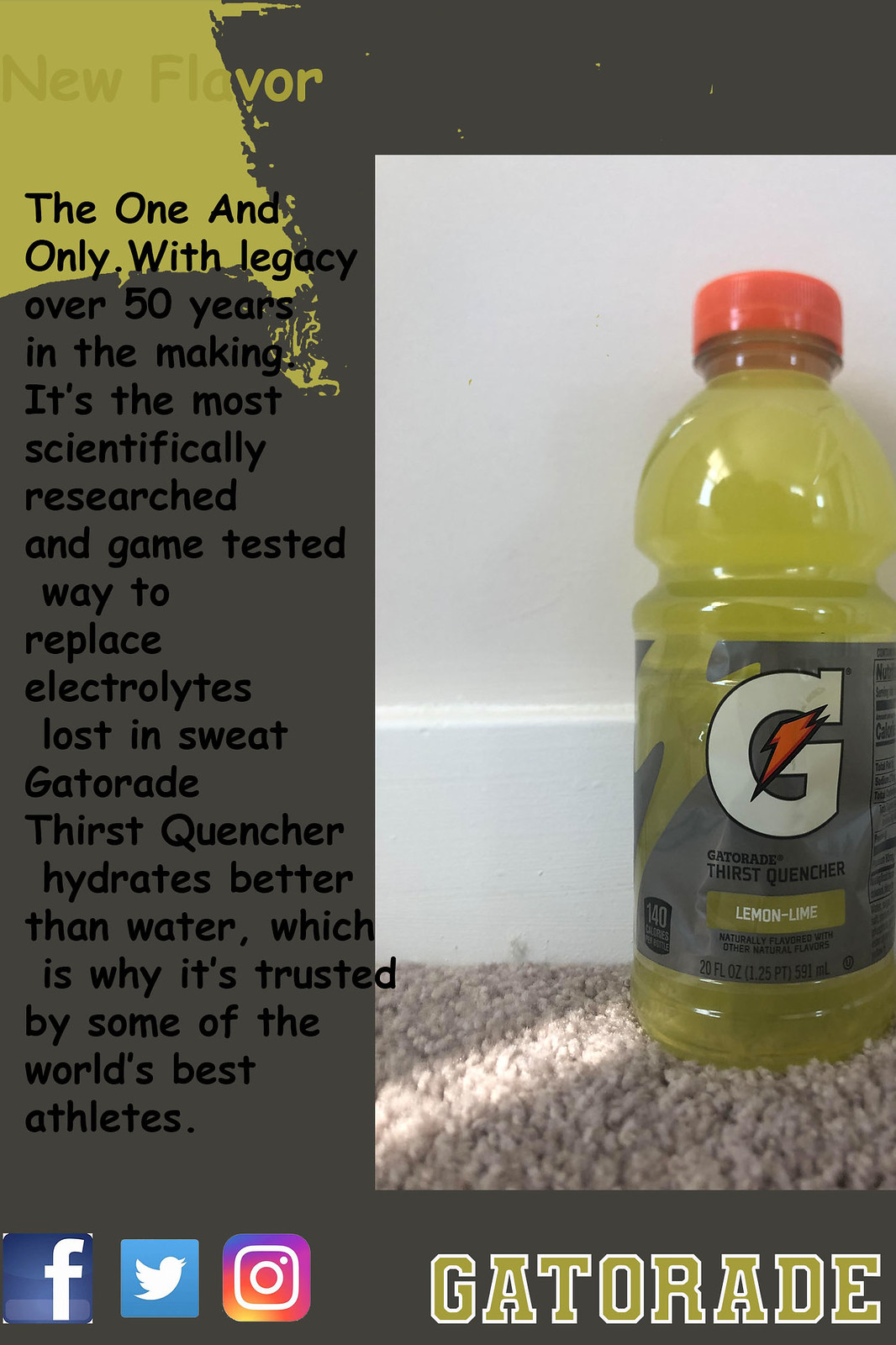The advertisement poster for Gatorade features a comprehensive and dynamic design that is primarily set against a light olive green and grey background. Dominating the right side of the poster is a striking image of a yellow Gatorade bottle with an orange cap, wrapped in a grey label boasting a large white "G" for Gatorade. Yellow text at the top left announces a "new flavor," while below, in black text, it proclaims: "The one and only with a legacy over 50 years in the making. It’s the most scientifically researched and game-tested way to replace electrolytes lost in sweat. Gatorade Thirst Quencher hydrates better than water, which is why it’s trusted by some of the world's best athletes." The word "Gatorade" appears prominently in yellow text with a white outline, using a sporty font. The bottom left corner features icons for Facebook, Twitter, and Instagram, indicating its presence on social media.